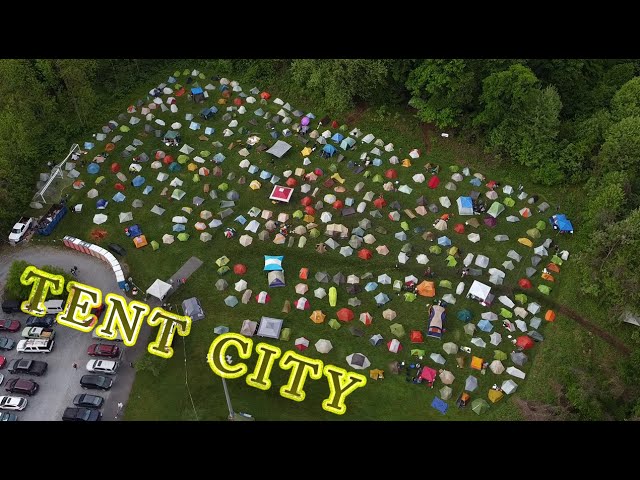An aerial photograph captures a sprawling campground from several hundred feet in the air, likely taken from a drone. The image reveals a vast green grass field teeming with over 100 small tents of various colors—reds, blues, whites, greens, and grays—appearing as mere dots from this height. The vibrant tents create a patchwork of color beneath the forest canopy that surrounds the entire site. On the left side of the image, a large blue trash receptacle is visible. 

Adjacent to the field, on the bottom right corner, lies a parking lot filled with more than a dozen cars, including SUVs, hinting at the photograph's recent origin. A curving roadway runs from the lower left and loops around, bordered by a row of approximately a dozen port-a-potties near the parking area. Additionally, the phrase "Tent City" is inscribed in two words at the bottom corner of the image in dark letters with a neon yellow outline, completing this detailed overview of the bustling encampment.